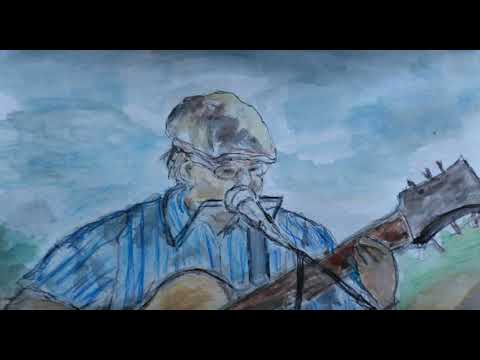This wide rectangular image displays a detailed drawing, framed by thick black borders at the top and bottom. The artwork, possibly created with watercolors or colored pencils, captures a serene scene with a cloudy sky filled with shades of blue, white, and gray, and a horizon that blends into tones of green and brown. The central figure is an older gentleman, visible from the shoulders up, playing an acoustic guitar with a light brown body and a dark brown neck.

He wears a short-sleeved, collared shirt with vertical stripes in various shades of blue, accented with hints of white. Upon his head rests a gray newsboy cap, and circular glasses perch on his nose. His hair, slightly disheveled, peeks out from under the cap. Positioned before him is a microphone, suggesting he is in the midst of a performance. Additionally, a harmonica, held up by a metal mouthpiece, is partially visible in front of his mouth. His left hand is seen fingering the guitar strings, while the right hand, presumed to be strumming, is out of frame. This intricate depiction captures a moment of musical expression, offering a glimpse into the man's passion and artistry.